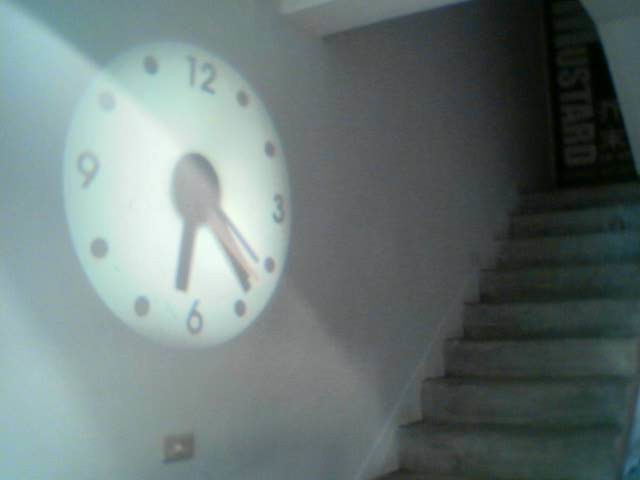In this photograph, a clock image is boldly projected onto a pristine white wall, casting a luminous display across the surface. The projection creates a bright spot in the bottom left corner, giving it a subtly enhanced glow compared to the rest of the dimly-lit room. The wall stands adjacent to a staircase, which is covered in a cozy gray carpet leading upwards. At the top of the stairs, a door marked with the word "MUSTARD" in white letters catches the eye, adding an intriguing focal point. The projected clock itself features a minimalist design with a white face, adorned only by the numerals 12, 3, 6, and 9, while the remaining hour positions are marked by simple circular dots. The time displayed is 6:24, indicated by bold black hour and minute hands, and a striking orange second hand that adds a pop of color to the monochromatic palette.